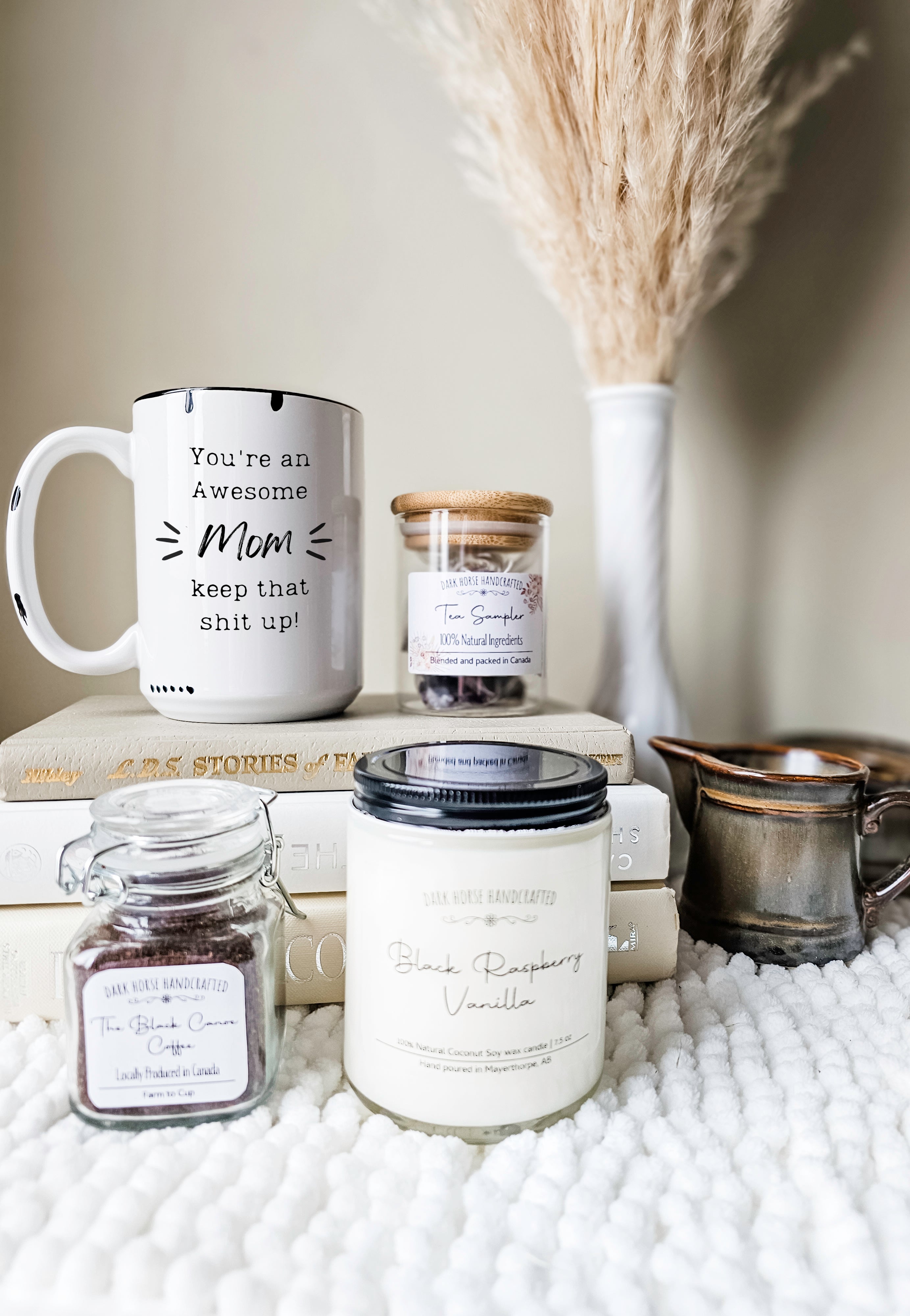The image, seemingly from a designer's website or social channel, captures an elegantly styled interior scene. Centered on a plush, fluffy, white mat or possibly a couch or ottoman, the photograph artfully showcases a serene still life arrangement. At the forefront, there's a small coffee jar and a black-lidded candle labeled "Black Raspberry Vanilla." Behind these items stand three stacked, neutral-toned books. Atop the books, a white mug, which appears aged with a peeling paint effect, boldly declares, "You're an awesome mom, keep that shit up!" with an exclamation mark. To the right of the mug sits a small glass tea jar with a wooden lid labeled "Tea Sampler." Complementing the scene, a light brown pottery creamer and a white vase filled with tan, dried reeds add earthy touches. The harmonious blend of beige, white, cream, and brown hues creates a soothing and cohesive color palette, highlighting both the elegance and homeliness of the setup.